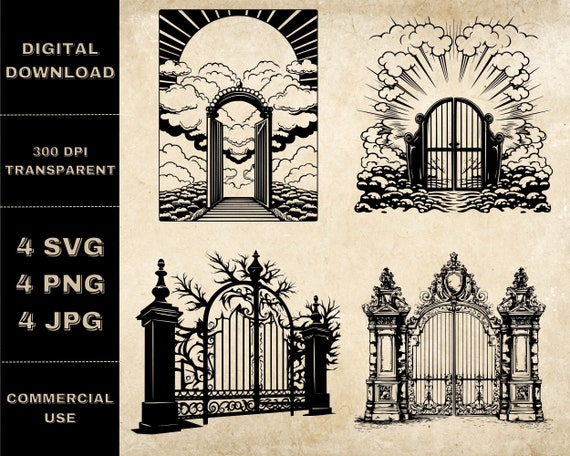The image depicts four detailed black-and-white illustrations of gates, laid out on a beige, worn-looking paper. On the left side, there is a black rectangular banner with white text that reads "Digital Download, 300 DPI Transparent, 4SVG, 4PNG, 4JPEG, Commercial Use." Each gate in the illustrations is unique and ornate. The top-left gate is arched and open, leading to a scene with an exaggerated sun and fluffy clouds, similar to a heavenly depiction. Cobblestone or a landscaped path adds detail to the scene. The top-right gate is closed and features wooden or metal slots, with a prominent doorknob, set against a backdrop of the sun beaming through clouds, giving an impression of a mystical or ethereal garden. The bottom-left gate appears vintage and wrought iron with intricate filigree and branches, flanked by ornately topped square columns. This gate gives off a slightly ominous vibe, reminiscent of an entrance to a haunted estate. The bottom-right gate is the most ornate, featuring rococo-style details and a crest, evoking the grandeur of a royal palace's entrance. All four images capture a blend of mystique and elegance, each telling a unique story through their detailed designs.